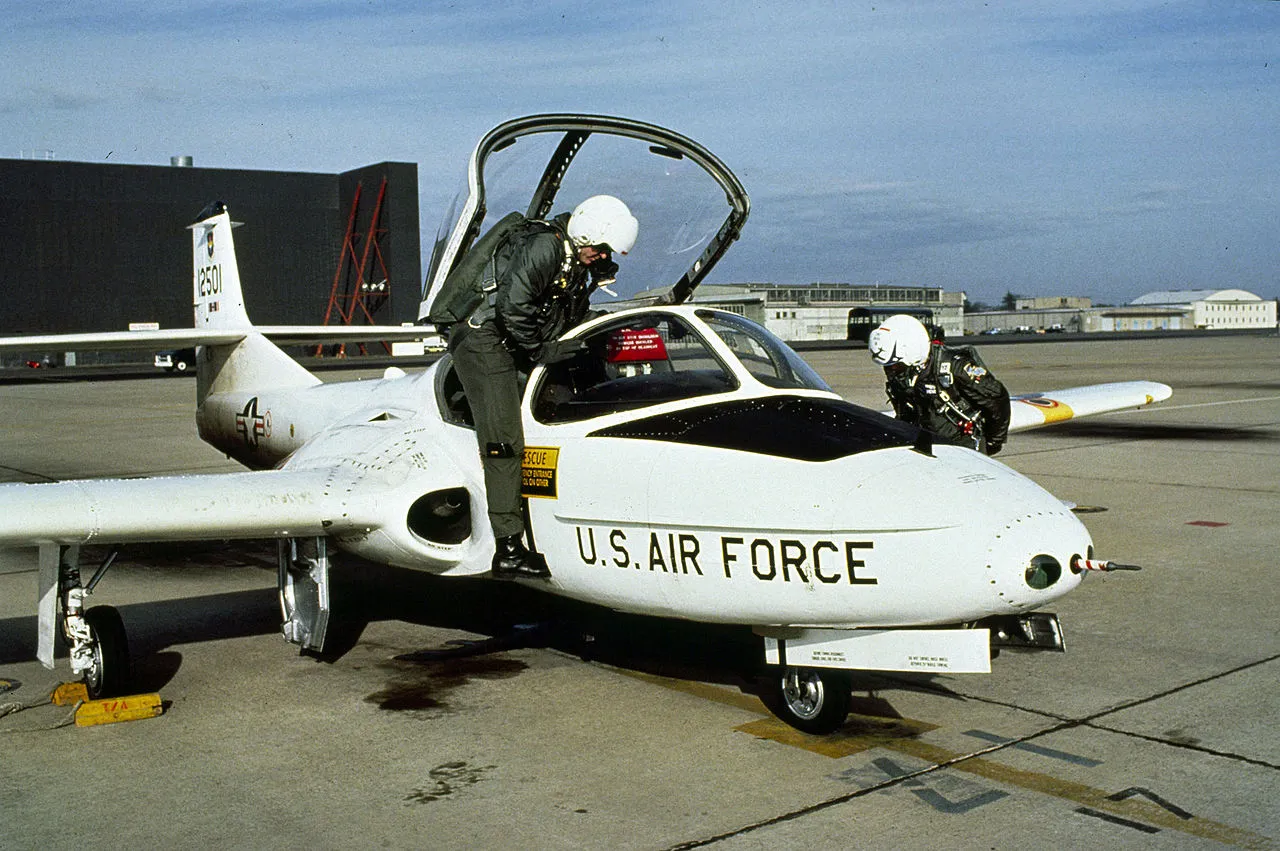The photograph captures a small white U.S. Air Force plane stationed on an airport runway. The aircraft, labeled with "U.S. Air Force" in black letters on its side and "12501" on its tail, sits low to the ground. Two men in black overalls with white helmets are interacting with the plane. One man, equipped with black shoes and a backpack (likely a parachute), is climbing into the passenger side, while the other man stands in front of the wings, examining the plane, possibly the engine, though it remains closed. A backdrop of a black building and several gray buildings stretch across the runway under a light blue sky stippled with soft clouds. The plane, positioned centrally with its nose pointing slightly to the right, is surrounded by the concrete expanses typical of air force bases. The scene features a palette of whites, blacks, grays, blues, and a hint of green.